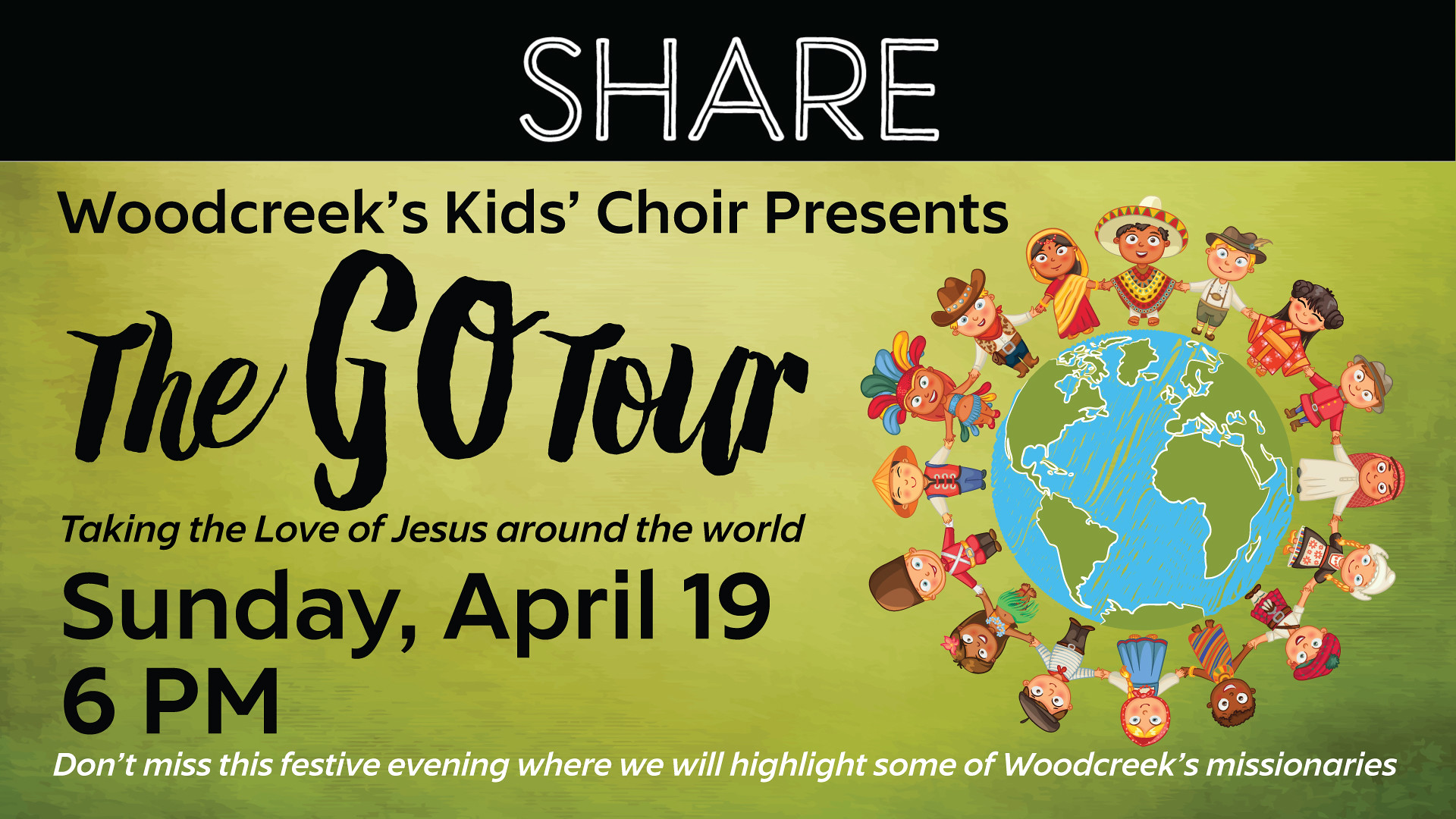The poster for Woodcreek's Kid's Choir Presents "The Go Tour" features a vibrant and inviting design. At the top, the word "SHARE" is prominently displayed in white letters on a black background. Below that, in black font, it reads "Woodcreek's Kid's Choir Presents" followed by "The Go Tour" in large script. The background transitions to a greenish color that occupies most of the poster. Dominating the right side of the image is a striking illustration: a blue globe with green countries, encircled by children holding hands, dressed in traditional outfits representing diverse cultures from around the world including Mexican, Indian, and American. Underneath "The Go Tour," it states "Taking the Love of Jesus Around the World," and provides the event details: "Sunday, April 19th, 6pm." The poster emphasizes not to miss this festive evening where some of Woodcreek's missionaries will be highlighted, adding a communal and celebratory touch to the announcement.